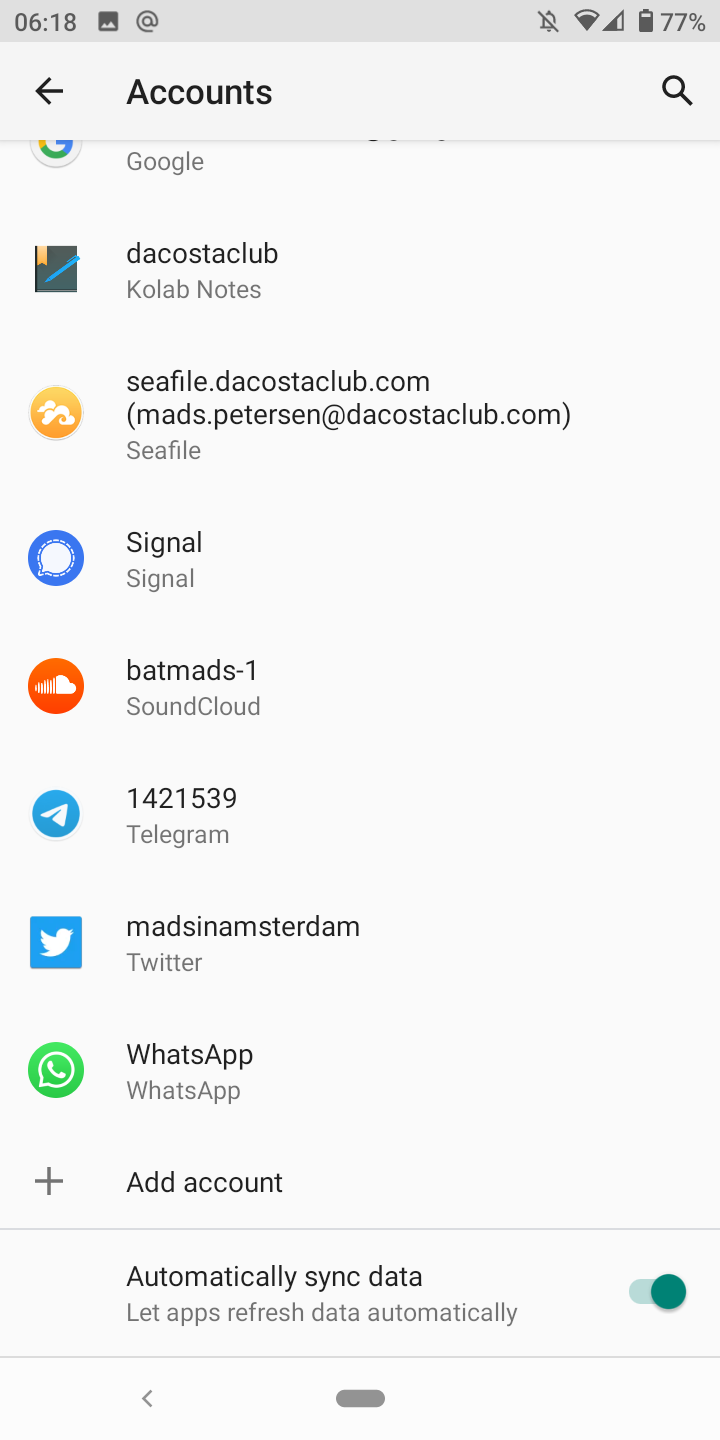The screenshot depicted in the image shows a smartphone screen. In the upper left-hand corner, the time is displayed as 6:18, while in the upper right-hand corner, the battery level is shown at 77%. Below this, the word "Accounts" is prominently featured. To the left of "Accounts," there’s a back button, and on the far right side, a search button is visible.

The main portion of the screen comprises a long list of various apps. At the top of the list, the Google app is partially cropped off. Below Google, the apps are listed as follows:
1. Da Costa Club
2. cfile.dacostaclub.com
3. Signal
4. batmads-1 SoundCloud
5. 1421539 Telegram
6. Mads in Amsterdam on Twitter
7. WhatsApp (indicated by its logo)

Further down, there is an option labeled "Add account." At the very bottom of the screen, the setting "Automatically sync data" is described with the subtitle, "Let apps refresh data automatically." This setting features an on/off switch, which is shown to be turned on in the screenshot.